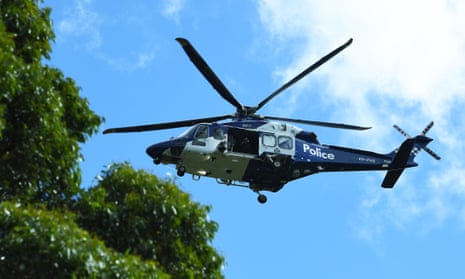The photograph captures a helicopter in mid-air, viewed from the ground, prominently centered in the image. This blue and white helicopter, marked with the word "POLICE" in white lettering on its tail, appears to have its door open. The helicopter's blue propeller and tail contrast with its white body. Surrounding the airborne vehicle, the background features a light blue sky with a large, fluffy white cloud situated in the upper right corner of the photo. To the left, there’s the top of a tree adorned with vivid green leaves, which exhibit a peculiar shine, adding a distinctive texture to the scene.